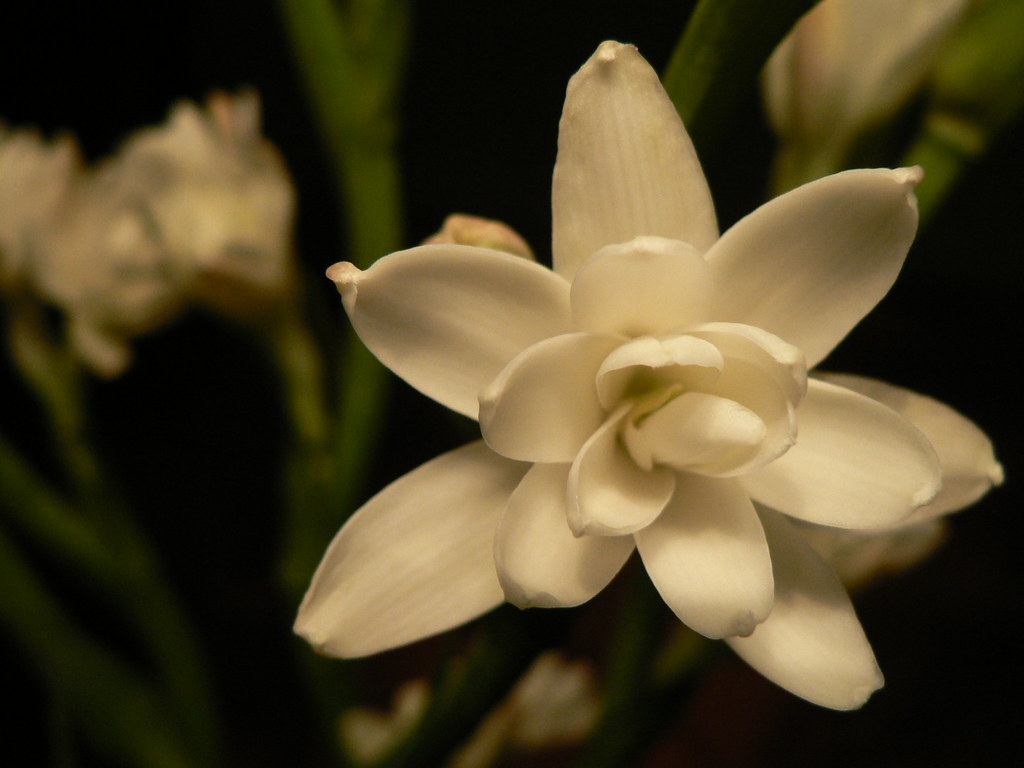In the close-up photograph, a stunning white flower dominates the right side of the image, extending from the center-left to the far right, occupying more than half of the frame. The flower showcases three distinct layers of white petals, with the outermost petals being long, thick, and oval-shaped, resembling magnolia petals. As the layers progress inward, the petals become rounder and smaller, forming a rosette pattern. At the very center lies a partially enclosed cone-shaped bud, possibly with a hint of yellow. The background is pitch black, making the flower stand out prominently. Blurry green stems emerge from the bottom, slightly left of center, and extend to the right, with additional unfocused white flower buds and stems visible, indicating other flowers yet to bloom.